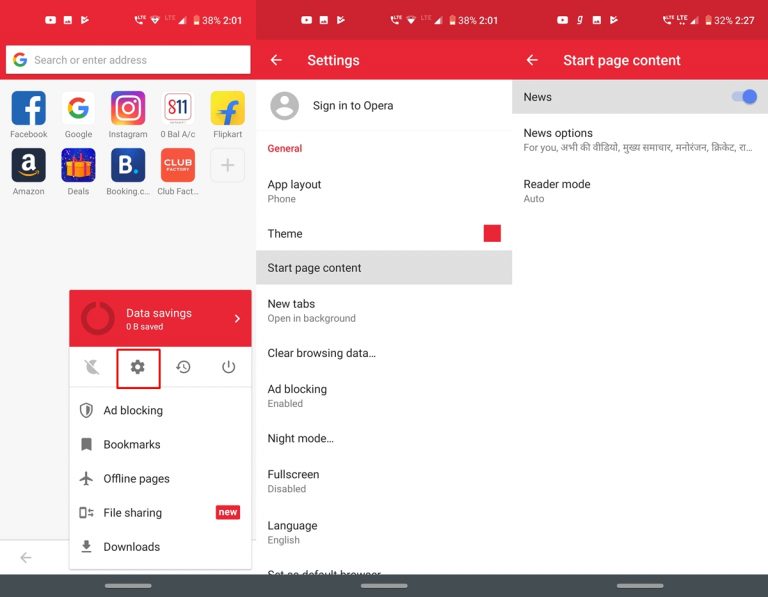This screenshot captures the interface of a desktop application, characterized by a dominant red theme. At the very top, there is a bright red banner followed by a dark red banner. Below this is the Gurgle logo accompanied by a search bar labeled "search or enter address." Another bright red banner appears underneath it, displaying options such as "Settings" and "Go Back."

On the right side of the interface, under the "Settings" heading, there's a "Go Back" button followed by "Start Page Content." Vertically listed along the left side under the search bar are several recognizable logos: Facebook, Google, Instagram, Zero Ball AC, Flipkart, Amazon, Deals, Booking.com, Club Factory, and a plus sign.

Toward the bottom of this list is a red banner indicating "Data Savings 0.8 saved," accompanied by a forward button. Further down are buttons for "Night Mode," "Settings" (highlighted with a red block), "Time," and "Power Off." Below these are options for "Ad Blocking," "Bookmarks," "Offline Pages," and "File Sharing." Adjacent to these is another red box with white text labeled "New," positioned above the "Downloads" box.

To the far left, more options appear including "Sign in to Opera" and "News."